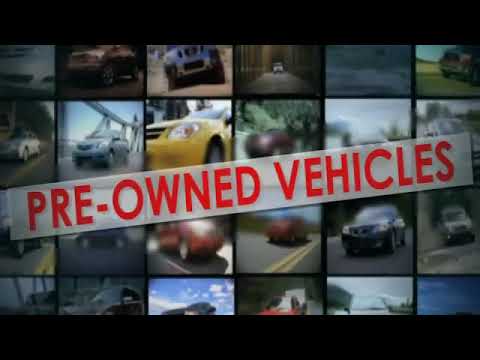The image is a collage of 24 square pictures showcasing various types and colors of vehicles, positioned in a grid of six across and four down. The vehicles include yellow, red, blue, white, and silver cars, as well as SUVs and Jeeps, though some of the images are partially shown or blurry. A white tape with the words "Pre-Owned Vehicles" printed in red runs diagonally across the image from left to right. At the center of the collage is a prominent yellow vehicle, with a red one directly below it. The top left picture features a white vehicle, while the bottom right image shows a clear blue sky. The top and bottom edges of the image are black, giving it a framed appearance. Overall, the collage appears to be an advertisement or a still from a video, emphasizing the variety of pre-owned vehicles available.